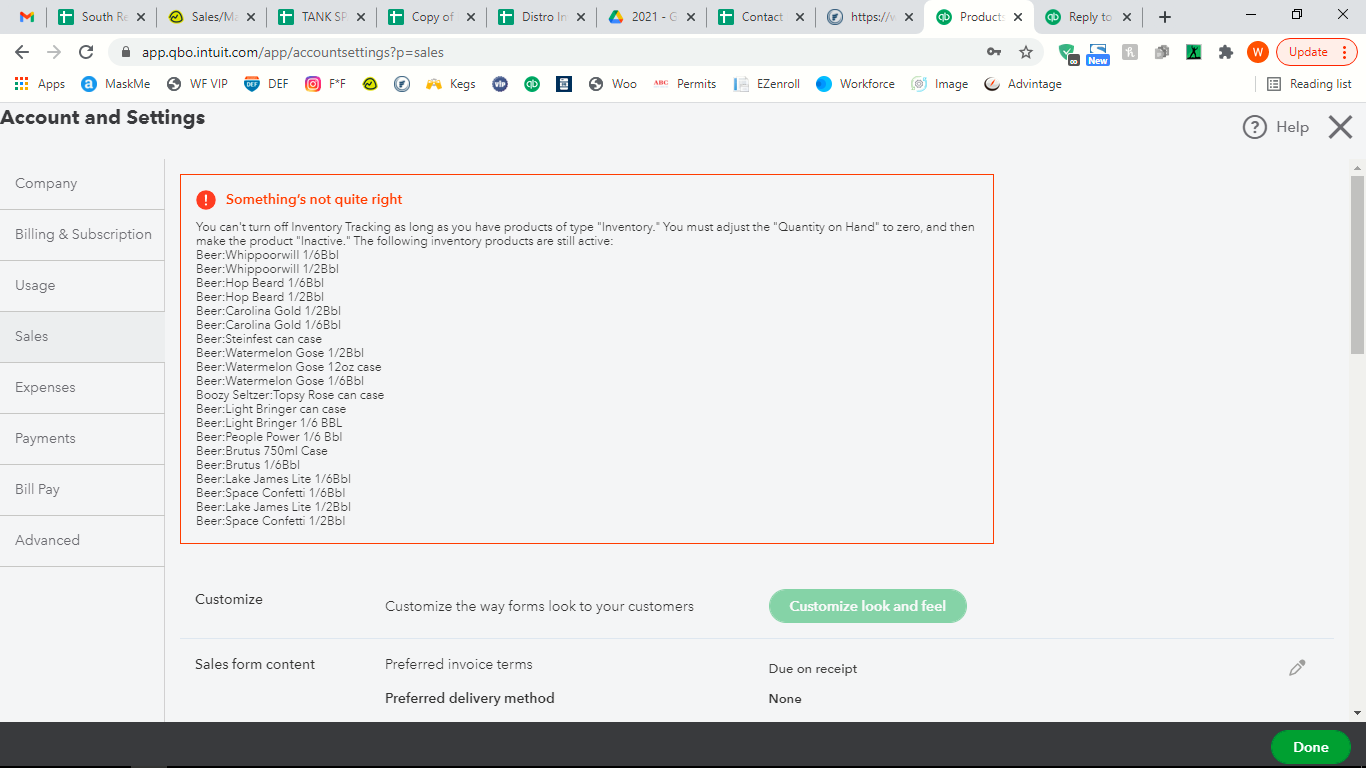The image displays a laptop monitor with ten open browser tabs, showcasing a busy digital environment. The active tab is on Intuit.com, specifically the QuickBooks Online (app.qbo.intuit.com) Account Settings page. The settings categories listed from top to bottom include Company, Billing and Subscription, Usage, Sales, Expenses, Payments, Bill Pay, and Advance. A Google icon is situated in the top left corner of the screen. A "Done" button appears in the bottom right corner. A dark gray to black banner spans the bottom of the image. In the upper right corner, there is a pink "Update" button for the web browser, indicating that an update is available.